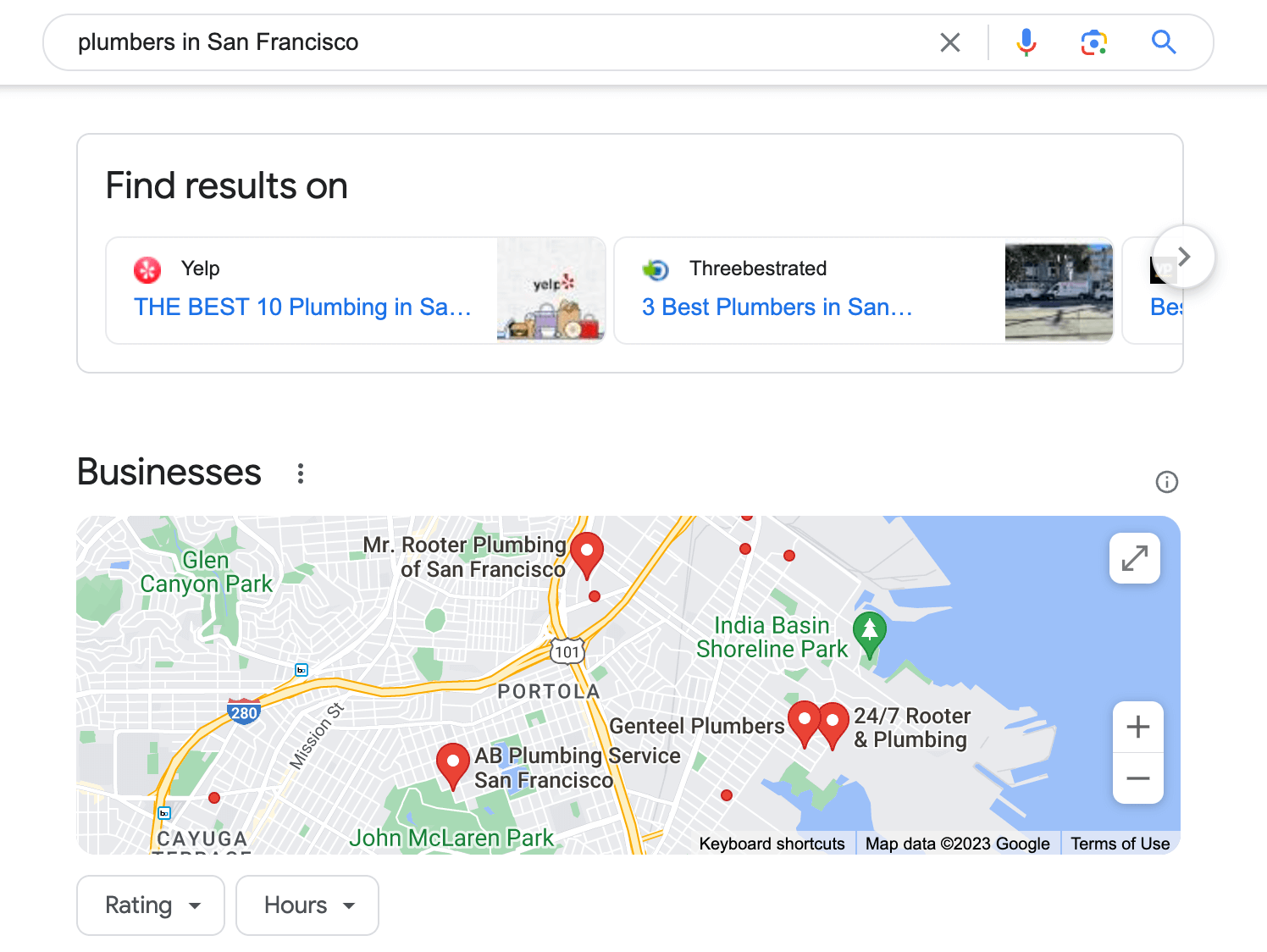The image is a screenshot of search results found online, displayed on a white background. 

At the top of the screenshot, there is a large search box spanning from left to right. It contains the text "plumbers in San Francisco," alongside an 'X' icon, a microphone symbol, a camera icon, and the traditional search magnifying glass.

Below the search bar is a section of search results within a rectangular box. This box is divided into two main sections. The first section, positioned to the left, showcases search results from different websites. The top result is from Yelp, identified by its red and black logo. The partial title reads "the best tin plumbing in SA," accompanied by a small Yelp photo-icon hinting at photo packages. The second result is from a site called "Three Best Rated," distinguished by a blue and green circular logo. The text reads "three best plumbers in San Francisco," next to an outdoor-themed, though indistinct, photo.

Adjacent to this, on the right, there is a box dedicated to physical business listings accompanied by a map. This map highlights several plumbing businesses within San Francisco. Notable entries include Mr. Rudder Plumbing of San Francisco, AB Plumbing (San Francisco), Gentile Plumbers, and 24-7 Rudder Plumbing. The map indicates that these businesses are situated between India Basin Shoreline Park, Glen Canyon Park, and John McLaren Park, suggesting they are within close proximity to one another. The businesses are marked with familiar red location arrows, commonly seen in such search interfaces.